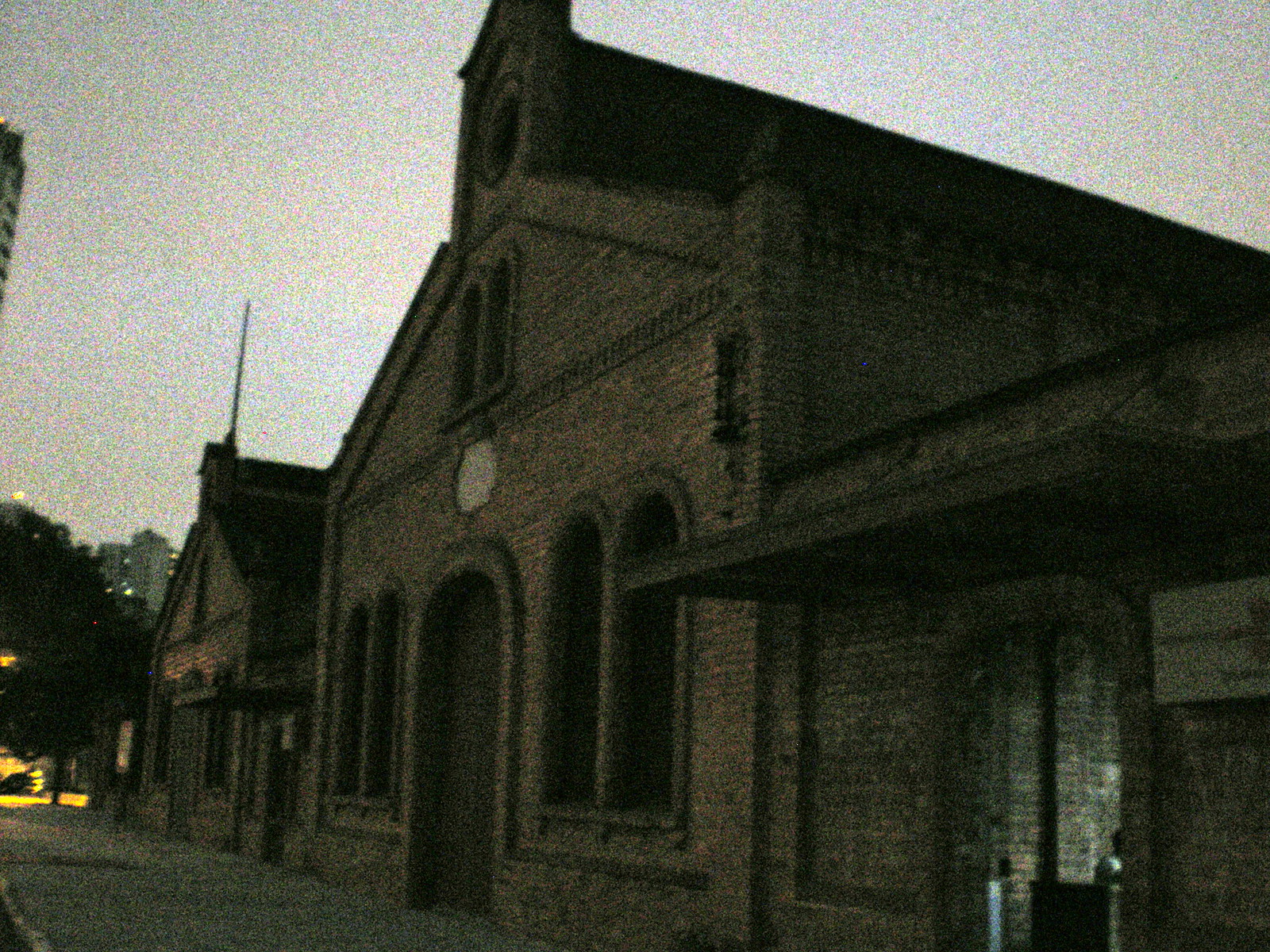This grainy photograph captures the solemn beauty of a crumbling, old brick church situated in an urban area at dusk or early dawn. The building, with its distinctive brownish-reddish stone bricks, features a rounded door at the center flanked by two arch-topped windows. Higher up, another pair of rounded windows sits beneath a deteriorating steeple, hinting at its past grandeur. Despite the ruinous state, where bricks are visibly falling, the structure stands testament to a bygone era, seemingly abandoned for a considerable time. In the foreground, an aged, expansive sidewalk leads to the church, while a towering tree stretches towards the sky at the far end of the building. The cityscape in the background reveals high-rise buildings, potentially 25 to 30 stories tall, casting faint, distant light against the grainy, bright white sky.